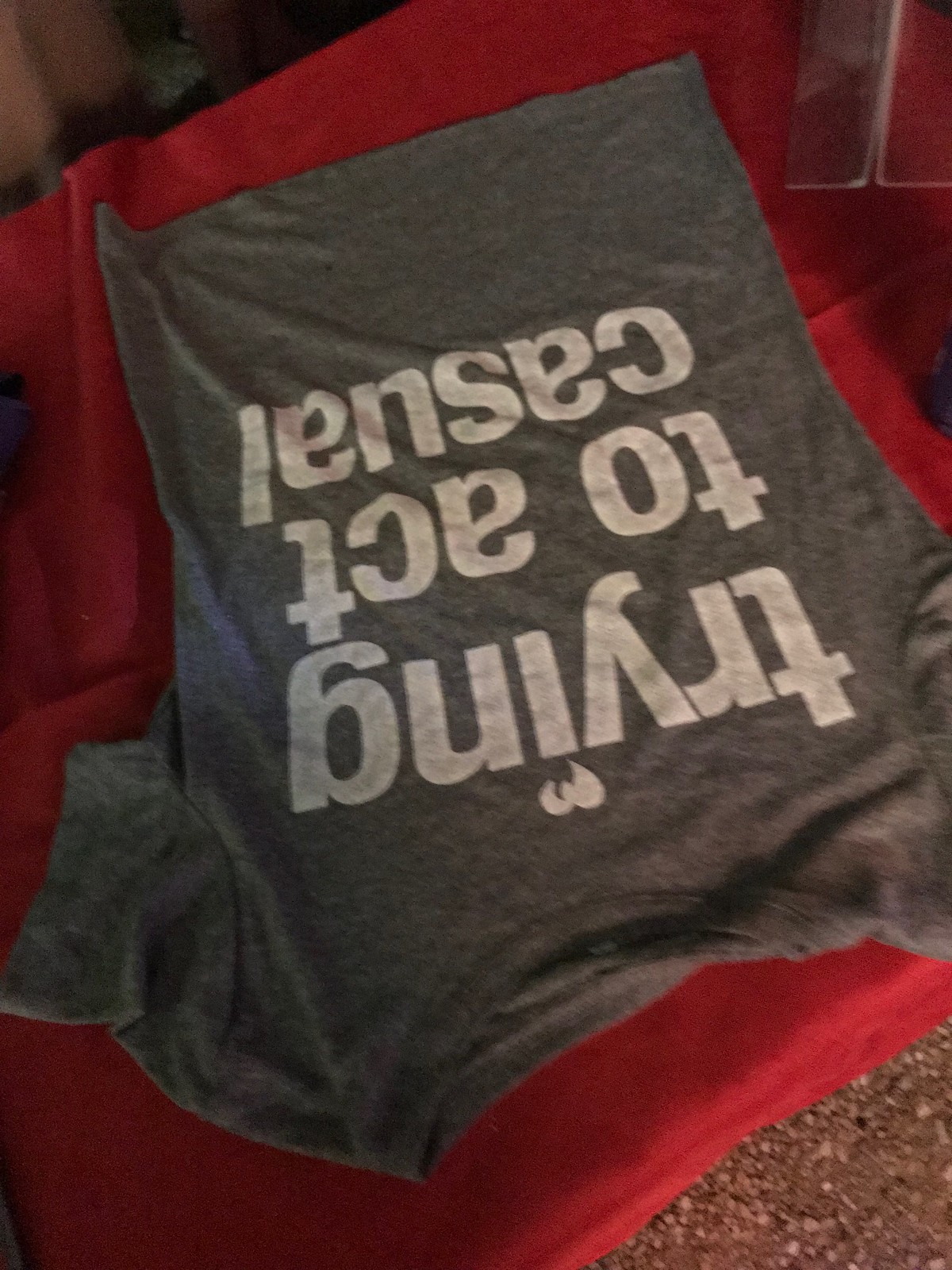The image depicts a slightly worn, gray T-shirt with some wrinkles. The T-shirt features an upside-down white print stating "Trying to act casual," with a stylized heart or flame-like design over the "i." This gray T-shirt is laid out with its sleeves spread and sits atop a red piece of fabric, possibly a folded shirt or tablecloth. The background consists of a reddish concrete surface with white stone inclusions, giving it a rough texture. In the upper right-hand corner, there is a barely discernible, transparent plastic card. The upper left-hand corner of the image is dark and indistinct, possibly showing a gray object against a brown background. The photograph itself is slightly blurry, giving it an amateurish feel, suggesting it could be an image intended for a sales listing.